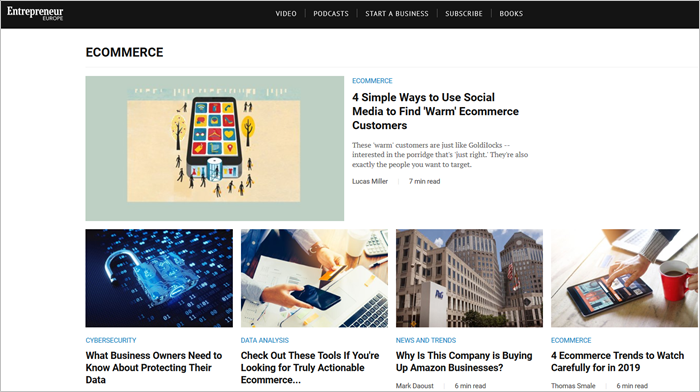Certainly! Here's a cleaned-up, detailed caption for the described image:

---

The cover of "Psycho Entrepreneur" magazine showcases a dynamic interface blending cutting-edge tech and business insights. The webpage is designed with a modern aesthetic, featuring a white background and a black navigation bar at the top with white text that includes categories such as Videos, Podcasts, Start a Business, Subscribe, and Books. The central theme on display is e-commerce, with an article titled "Four Simple Ways to Use Social Media to Find 'Warm' E-commerce Customers" headlining the page. 

The visual centerpiece is a striking computer-generated image of a monumental smartphone surrounded by bustling virtual figures, symbolizing the magnetism of social media in attracting the ideal customers—those who are 'just right', akin to Goldilocks' perfect porridge. Below this, additional articles cater to the astute entrepreneur, covering critical topics like "What Business Owners Need to Know About Protecting Their Data", illustrated by an image of an open padlock, and "Check Out These Tools If You're Looking for True Interaction in E-commerce", featuring a businessman engrossed in his laptop and smartphone amidst a busy urban backdrop.

Another notable feature is a story on the acquisition trends titled "Why This Company is Buying Up Amazon Businesses", juxtaposed with a serene cityscape shot. Finally, the section closes with "Four E-commerce Trends to Watch Carefully For in 2019", accompanied by an image of a woman multitasking—holding a tablet in one hand and a coffee cup in the other—capturing the spirit of the modern e-commerce professional.